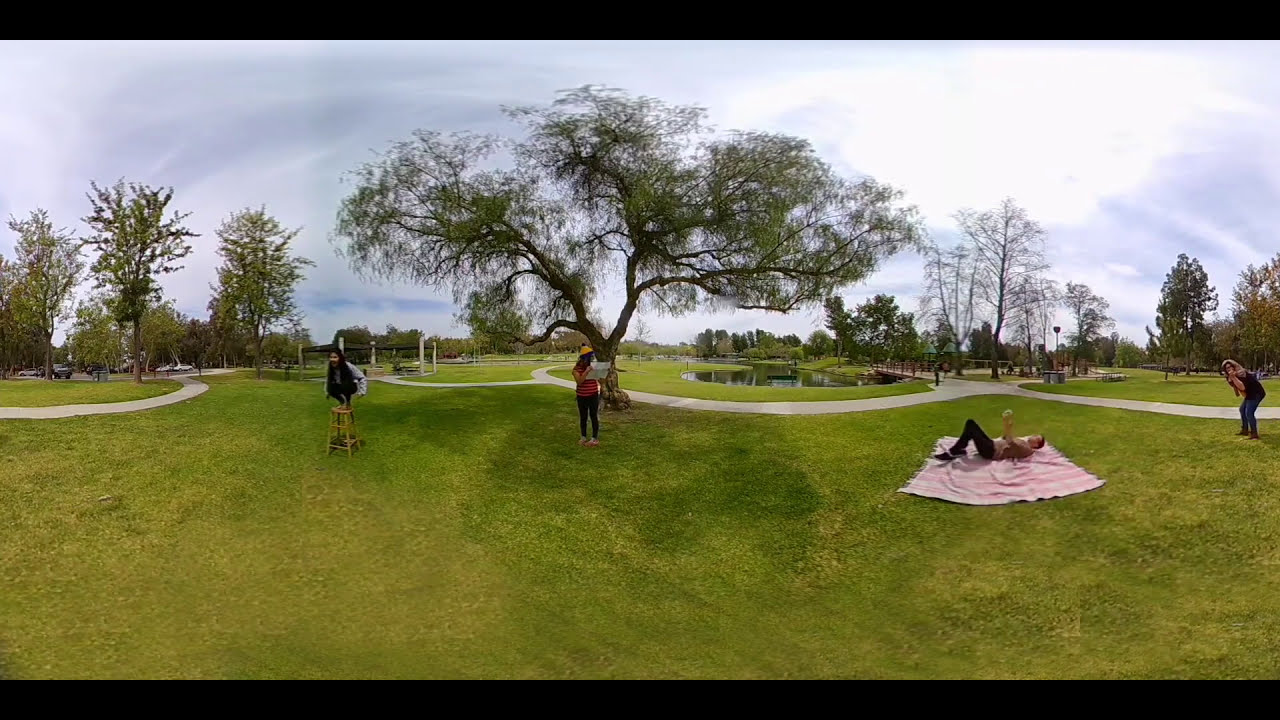The image depicts a lively scene in a park with four individuals engaged in various activities. On the grass, a man reclines on a pink and white picnic blanket, his knees bent and arms raised, dressed in black trousers and a brown shirt. Centered in the frame, a woman in an orange and red striped shirt with black trousers and a yellow beanie is holding up and reading a piece of paper. She stands in front of a small, wide tree, looking to her right. To the left, a person with long black hair and a white jacket squats on a wooden stool. In the right-hand corner, another individual, bent over with their knees slightly bent, appears to be taking a photograph of the scene, hands raised to their face. The park, blanketed with short green grass, features a winding concrete path, a plethora of large trees, and a background that includes a pond, playground, and some out-of-focus structures like a car park. The image, taken during the day under a relatively cloudy sky, showcases a peaceful yet vibrant outdoor environment.